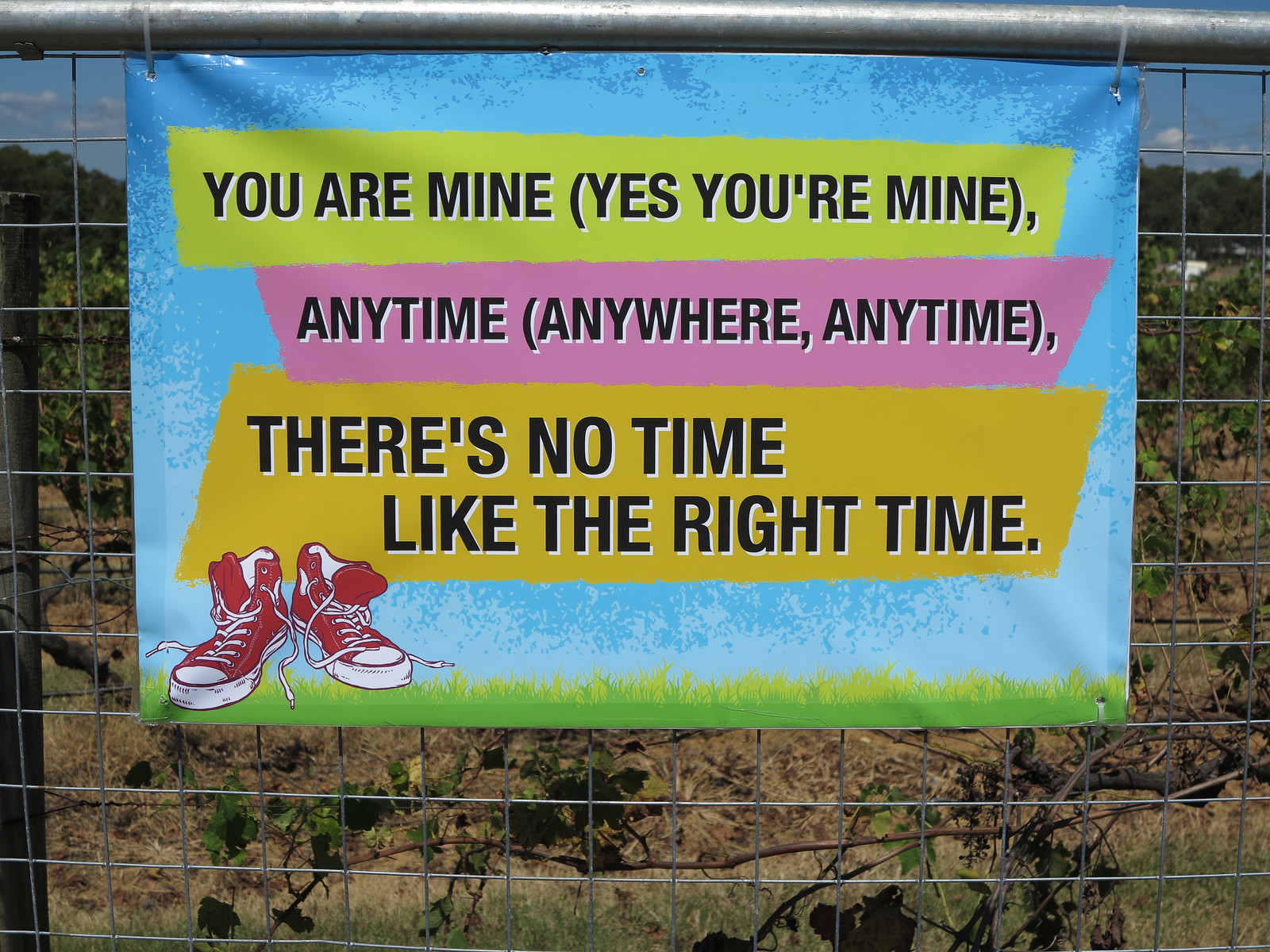This outdoor image features a banner hanging from the horizontal post of a metal fence, characterized by square wire holes. The banner stands out with its vibrant blue background and text in black with a white drop shadow. The message reads: "You are mine, yes, you're mine, anytime, anywhere, anytime. There's no time like the right time." The text is distributed across three color blocks—green at the top, pink in the middle, and a yellow-orange at the bottom.

An illustration of grass lines the bottom edge of the banner, adding a natural touch. In the bottom left corner, a pair of red high-top Chuck Taylor sneakers with untied, floppy white laces lie casually, suggesting they were just taken off. Behind the banner, the wire of the fence remains visible, with a backdrop featuring patches of green and brown grass, some low trees, vines, a building on the right, and larger trees further in the distance. The scene is capped off by a sky with puffy white and gray clouds, providing a serene and natural setting for the banner.